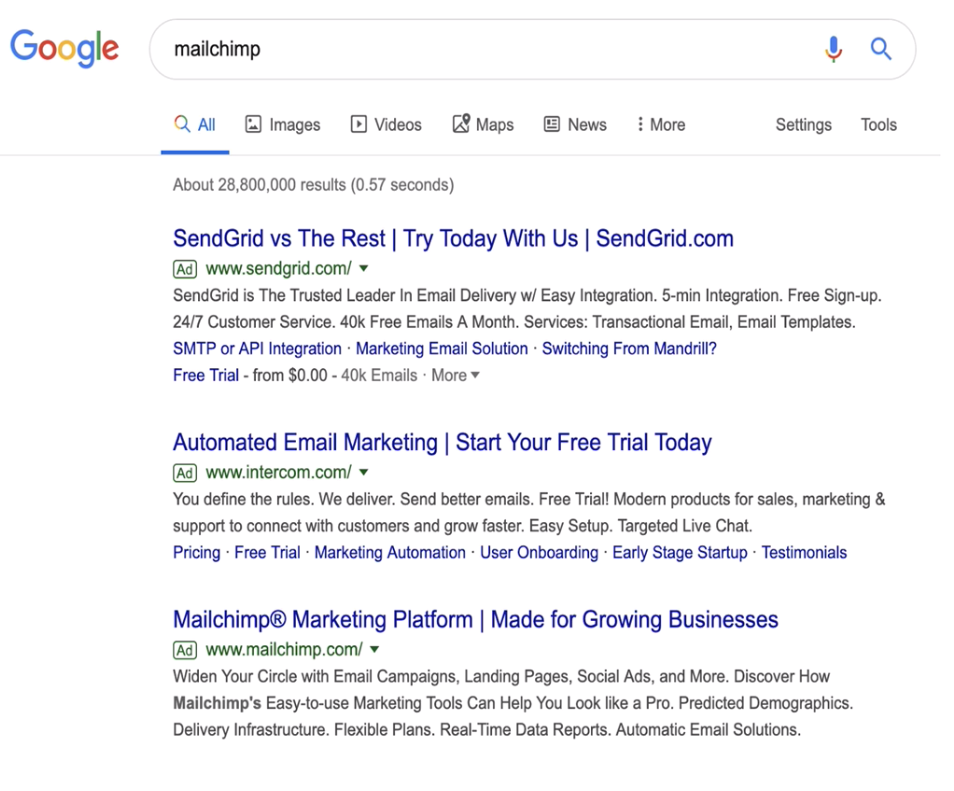The screenshot captures a Google search results page. In the upper left corner, the iconic Google logo is prominently displayed. To its right is a search field with the query "male chimp" entered. Adjacent to the search bar on the right, a blue microphone icon is visible, which allows for voice search, followed by a blue magnifying glass indicating the search button.

Directly under the search field, a row of filter options is presented, with "All" selected, as indicated by the blue font and underline. The other filtering options—Images, Videos, Maps, News, More—are in black font, while further to the right, Settings and Tools are also displayed.

Beneath the filters, in a darker font, the text indicates "About 28,800,000 results (0.57 seconds)" summarizing the volume and speed of the search query results. The actual search results begin right below this line.

The first result is an advertisement titled "SendGrid versus the rest. Try today for us, SendGrid.com," shown in blue font. Below it, the source URL is displayed in green with the label "ad" (www.SendGrid.com), followed by a brief description of the website content.

The second result is another advertisement for "automatic email marketing. Start your free trial today," again in blue font. It is identified as an ad by the green label next to the URL (www.Intercom.com), with subsequent descriptive text in black.

The third result continues in a similar format: "MailChimp marketing platform made for growing businesses" in blue font. Once again, it is marked as an ad, evidenced by the green ad label and URL (www.MailChimp.com), followed by additional descriptive text in black.